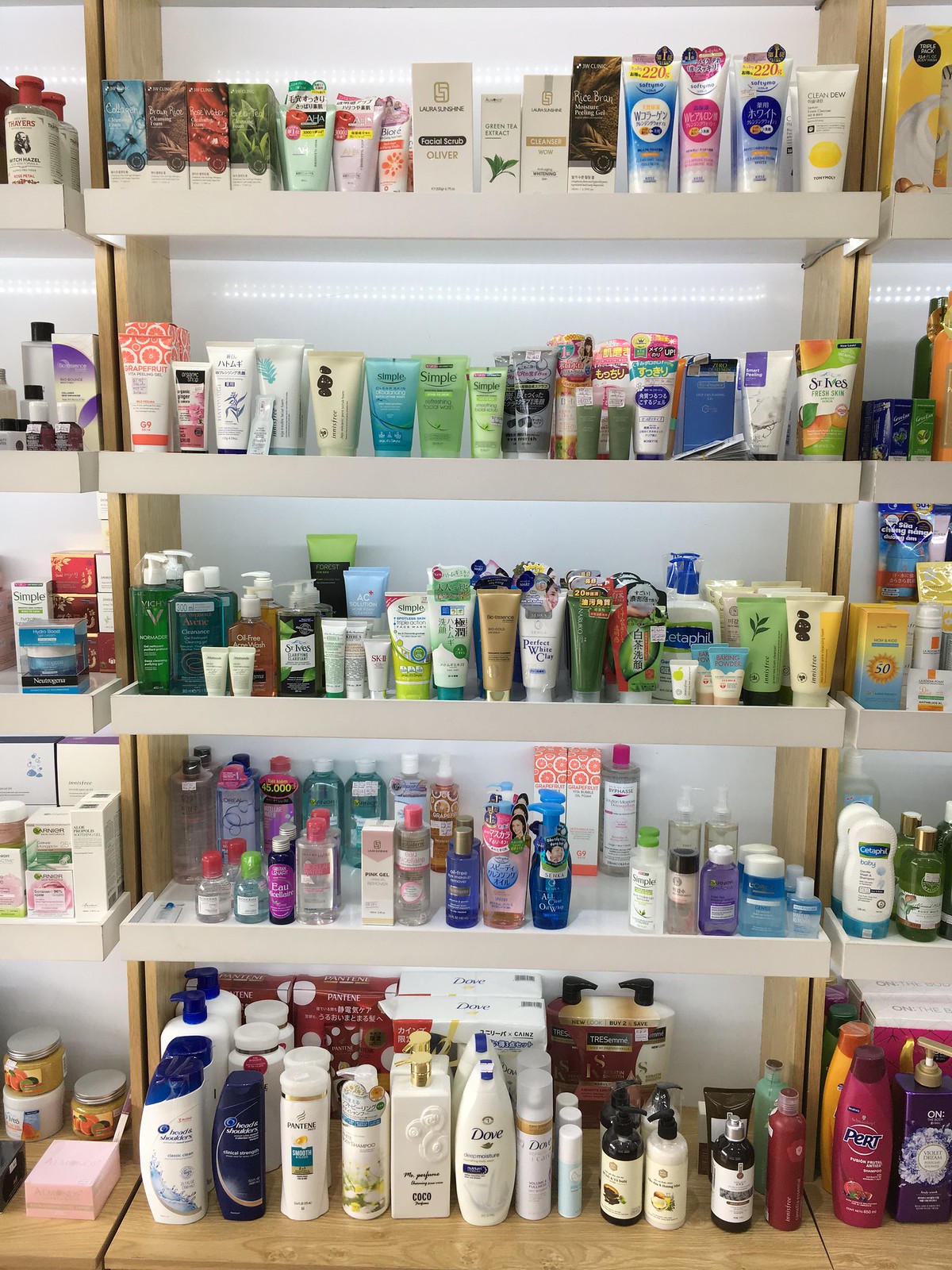The photograph depicts an aisle inside a well-lit drugstore, heavily stocked with a diverse array of skincare products. The shelves, which feature a lip to prevent products from falling, are supported by tan uprights and are themselves white. They are illuminated by overhead fluorescent lights, which reflect off a white wall behind, enhancing the visibility of the products.

The display consists of four shelves above a wood-colored surface. The shelves are filled with a variety of items, including tubes of lotion or sunscreen, which come in different shapes and sizes—some in boxes, some in squeeze tubes, each bottle varying in height. The assortment appears disorganized, with brands and products seemingly mixed together. Among the myriad of colors, one can spot hues of pink, bright blue, green, dark green, lime, coral, and aqua. Specific brands like Dove, Head & Shoulders, and St. Ives are visible, the latter featuring a squeeze tube with an apricot or peach design.

The image also shows parts of adjacent shelving units on both the left and right sides, which are cropped off. The products on these lower shelves include pump bottles, often used for lotions, while the higher shelves may contain boxes of soap. Overall, the scene is a vibrant mix of colors and product types, creating a visually engaging snapshot of the drugstore's skincare and shampoo aisle.